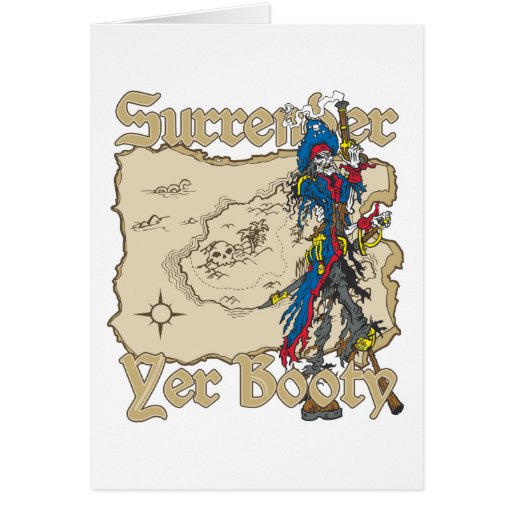This image depicts an opened greeting card resembling a postcard, standing upright against a white background. The card itself is white and features distinctively pirate-themed artwork on its cover. Across the top, in light brown text, the word "surrender" is prominently displayed, mirrored by the phrase "yer booty" at the bottom. Sandwiched between these texts is a detailed depiction of a pirate's map in a dusty, sand-brown color, complete with jagged edges. The map’s illustrations include various geographical elements like hills and islands, drawn in a darker brown, and whimsical features such as a compass, a Loch Ness Monster, and sketched trees and waves. Dominating the right-hand side of the map is a striking image of a deteriorated skeleton pirate dressed in vibrant blue, red, and yellow tattered attire, including a hat and pants. He holds a gun aloft, encapsulating the daring and rugged essence of pirate lore. This elaborate design, full of rich details, brings a classic pirate adventure to life on the card's surface.